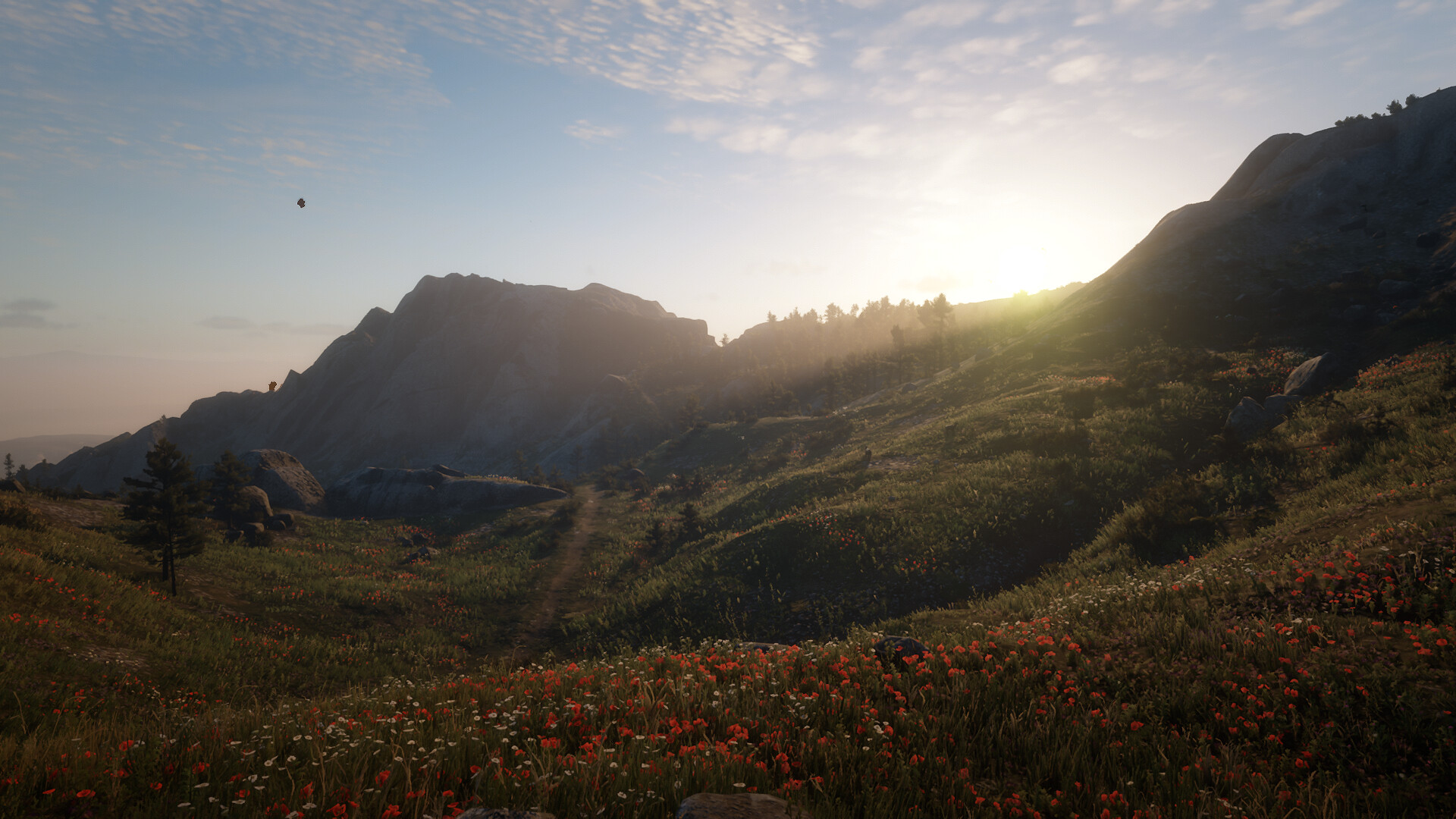This photo captures a picturesque meadow bathed in the golden light of the sunrise. The lush green ground is covered in abundant, vibrant grass, and the landscape gently undulates with rolling hills. The meadow is adorned with a sprinkling of red and white flowers, adding bursts of color to the verdant expanse. Scattered across the scene are small trees, though larger clusters are sparse.

A dirt road winds its way through the meadow, guiding the eye towards the towering, rocky mountains that dominate the distant horizon. These majestic peaks create a striking contrast against the bright, blue sky above. Puffy, cotton-like clouds are scattered throughout the sky, becoming thinner as they ascend. Near the horizon, clouds take on a soft pink hue, complementing the vibrant colors of the dawn. The entire scene exudes a serene and tranquil beauty, capturing the essence of a perfect morning in nature.